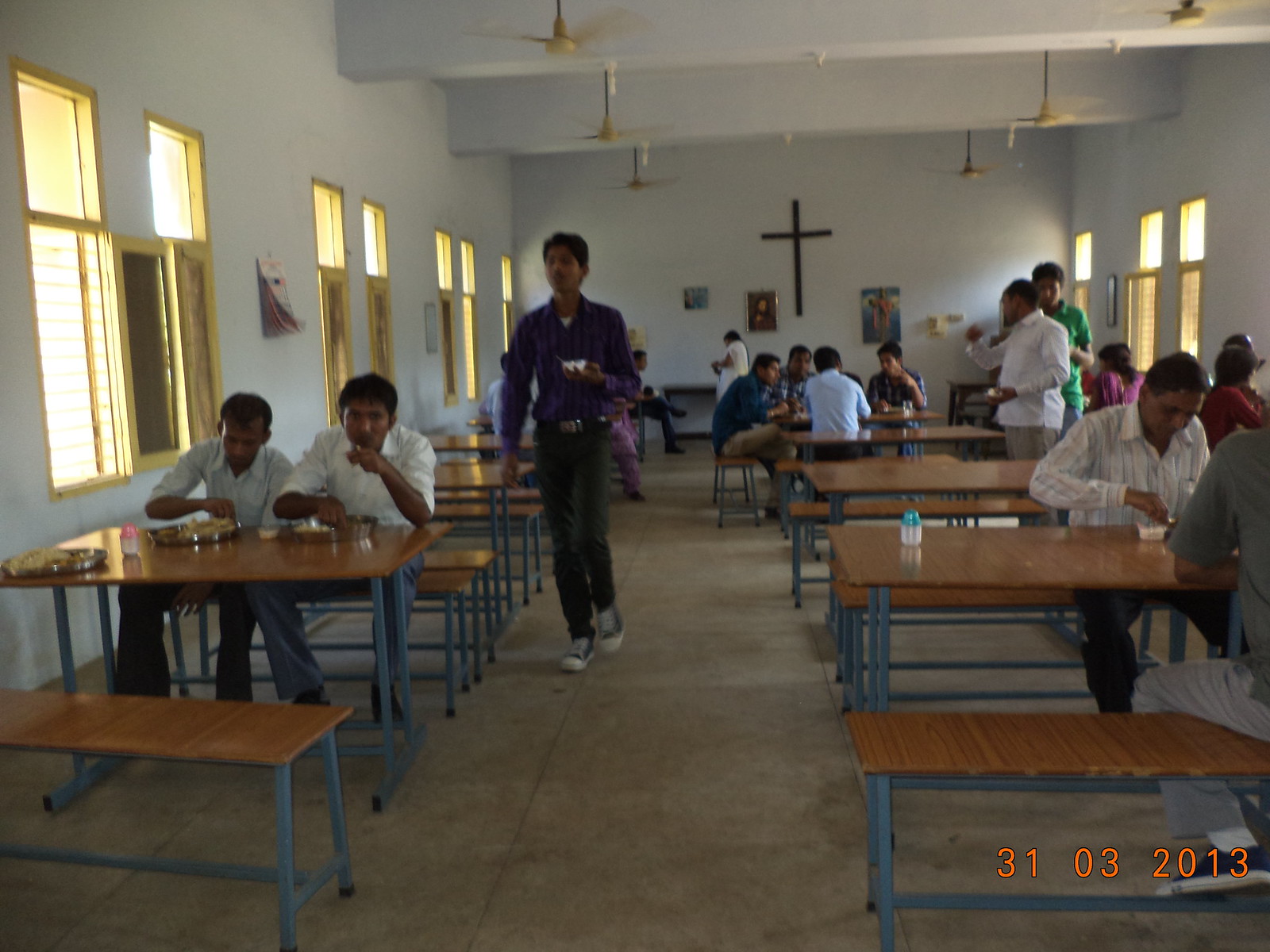This photograph, taken on March 31, 2013, depicts a communal cafeteria with a potential religious association, indicated by the black cross hanging on the back wall. The rectangular room features white walls and ceiling, beige floors, and uniformly lined up long windows on both sides, allowing yellow light to filter through yet keeping the interior dim. The space is divided into two columns of tables and benches with tan wooden tops and blue legs, sparsely populated by diners. In the foreground, two men in white button-down shirts sit at a table eating from metal containers, while a man in a purple shirt with black pants and sneakers walks between the tables holding a white vessel. The room also includes ceiling fans and several pictures, possibly religious in nature, further suggesting that this could be part of a church or a religious institution. The timestamp “3103 2013” is visible in orange font at the bottom right corner of the image.